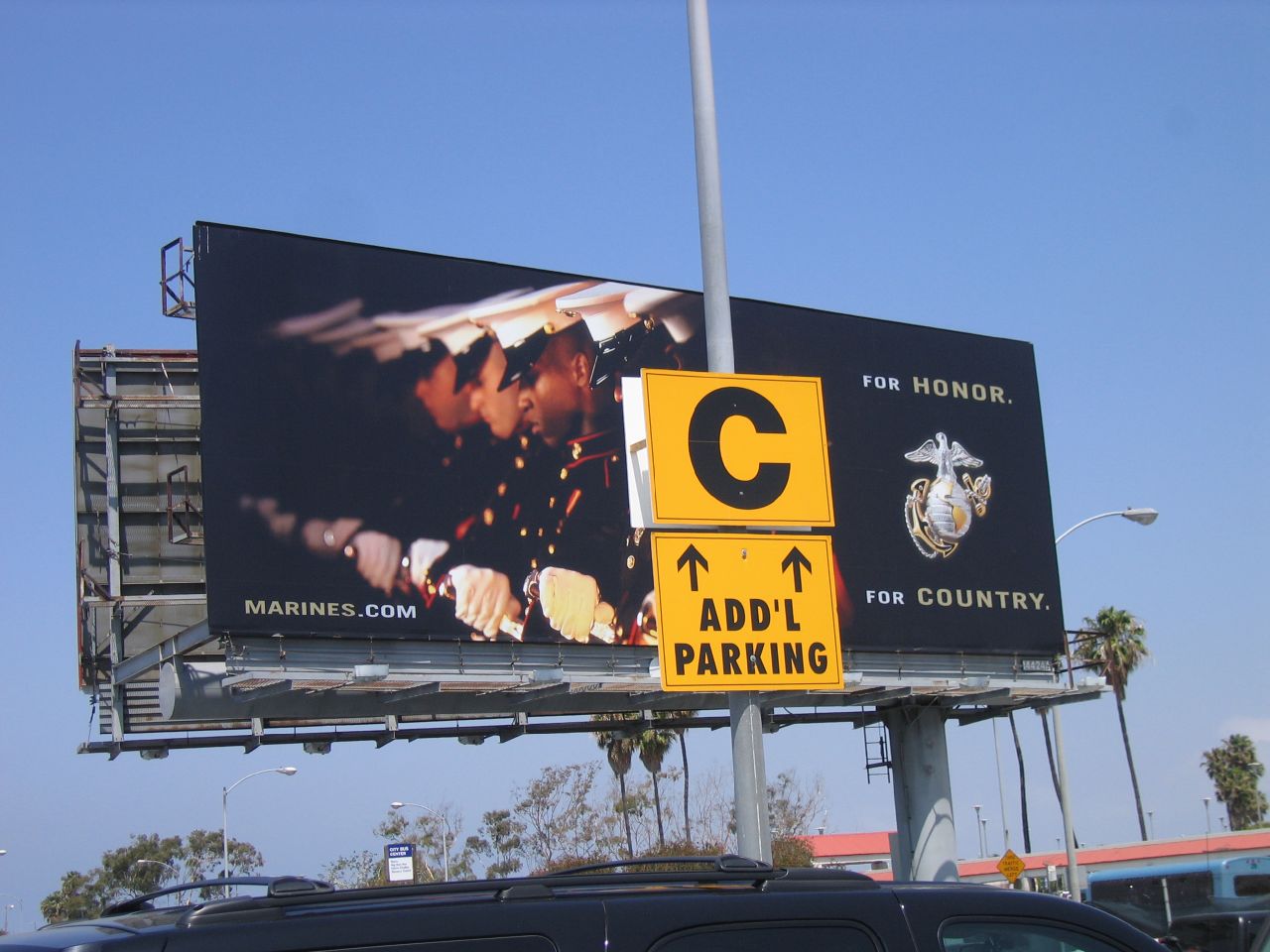This outdoor color photograph features a prominent billboard for the U.S. Marines against a backdrop of a clear, blue cloudless sky. The billboard, which dominates the scene, is flanked by palm and other green-leaved trees, and is situated along a roadside where the tops of vehicles are visible, including the roof of a dark blue or black SUV with roof racks in the foreground.

The billboard itself showcases a striking image of a row of male Marines in their dress uniforms, complete with white hats and gloves, all looking down in unison. This row is depicted from a side angle, approximately 31 degrees. On the left side of the billboard, the text "Marines.com" is displayed in white in the bottom corner. The right side features the Marine Corps emblem—a silver and gold insignia of an eagle, globe, and anchor—accompanied by the phrases "For Honor" in white and gold, and "For Country" also in white and gold.

Adding an additional layer to the composition, a pole stands in front of the billboard with two yellow signs: the top sign has a black 'C' on it, while the lower sign features two upward arrows and reads "ADDL Parking," indicating additional parking. The overall scene captures the prideful display of Marine Corps recruitment along with the practical signage for local navigation.